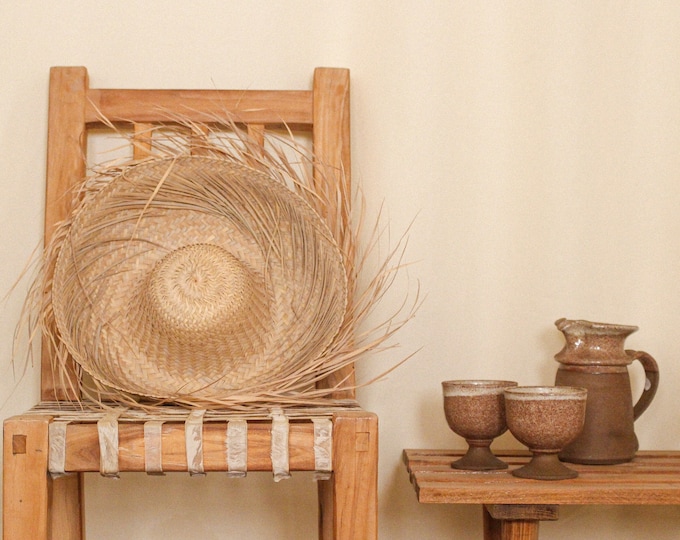The image depicts a room adorned with rustic decor. On the left, a wooden chair, featuring an interwoven lattice seat, sits against a beige wall. Atop the chair is a handmade straw hat with wisps of straw radiating outward, and the hat's brim appears unfinished. To the right of the chair stands a small, light brown wooden table, lower in height than the chair, which supports a stonewashed ceramic carafe with a large handle. Accompanying the carafe are two small, stoneware cups. The cups have rounded bodies that flare slightly at the bases, complementing the carafe in both style and material.